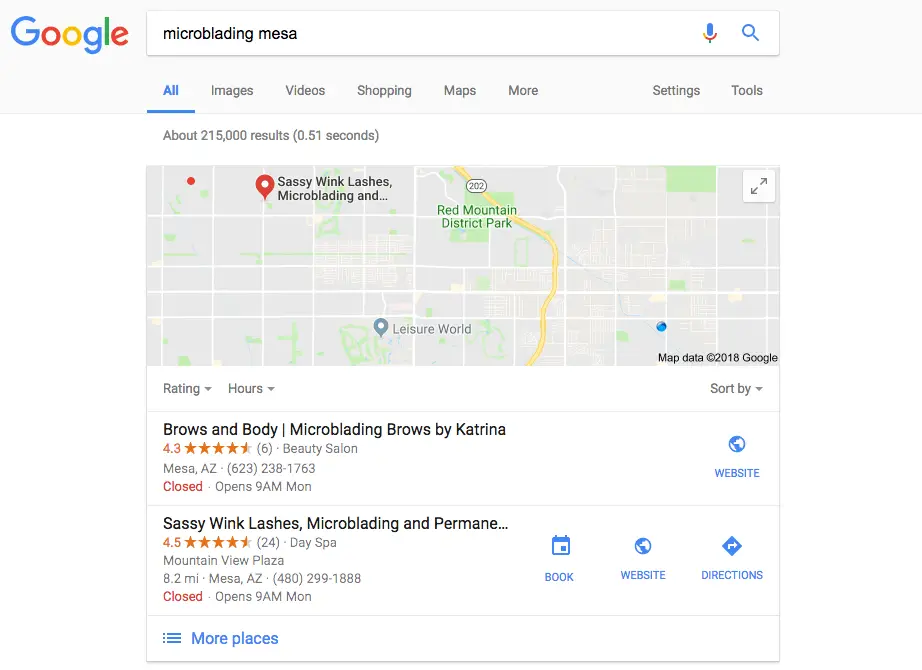This image is a detailed screenshot from a Google search, likely taken on a laptop, PC, or tablet due to its width, which is too broad for a mobile device. The background is light, and the iconic Google logo, sporting its familiar blue, red, yellow, and green colors, is visible in the upper left corner. The search term "microblading Mesa" is entered into the search box, and the "All" tab is selected, highlighted in blue among other filter options like Images, Videos, and Shopping.

Below the search box, there's a rectangular map featuring a red pin marking a business related to the search query. This business is named "Sassy Wink Lashes and Microblading." Further down, two relevant locations are listed. The first listing is for "Brows and Body - Microblading Brows by Katrina," which has a rating of 4.3 stars. It provides additional details like the location in Mesa, Arizona, the phone number, business hours, and a link to the website.

The second listing, corresponding to the pinned location on the map, is "Sassy Wink Lashes, Microblading and Permanent Makeup," which holds a rating of 4.5 stars. It's currently closed and will open at 9 a.m. Located in Mesa, Arizona, this listing also includes the phone number, and offers links to book an appointment, visit the website, and get directions.